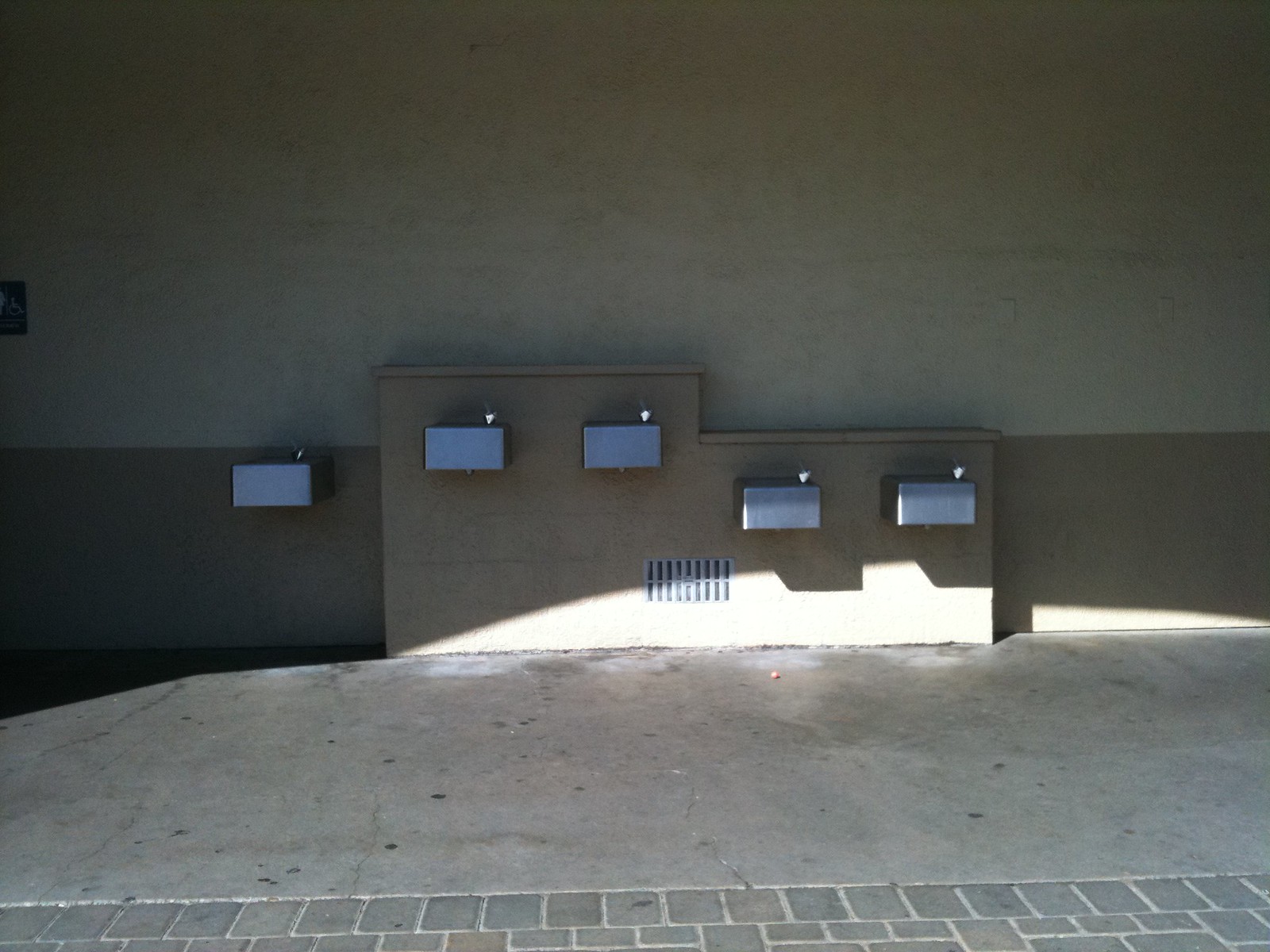The image depicts a two-toned wall, with a darker brown color at the bottom and a lighter tan above, partially illuminated by sunlight but mostly in shadow. In front of the wall, there is a gray concrete ground paved with square and rectangular stone tiles. Five silver metal drinking fountains are mounted on the wall; they are rectangular with drinking spouts on the right side. Two of these fountains are positioned at a lower height, suitable for children, while the other three are at standard adult height. Four fountains are grouped together in a staircase-like arrangement, with an additional fountain positioned separately to the side. A white vent is located at the base of the wall. A blue handicap sign featuring a white wheelchair icon is visible towards the upper left part of the wall. The setting resembles a bathroom area within a large cement building. A noticeable sign of wear on the ground is the presence of scraped-off gum.